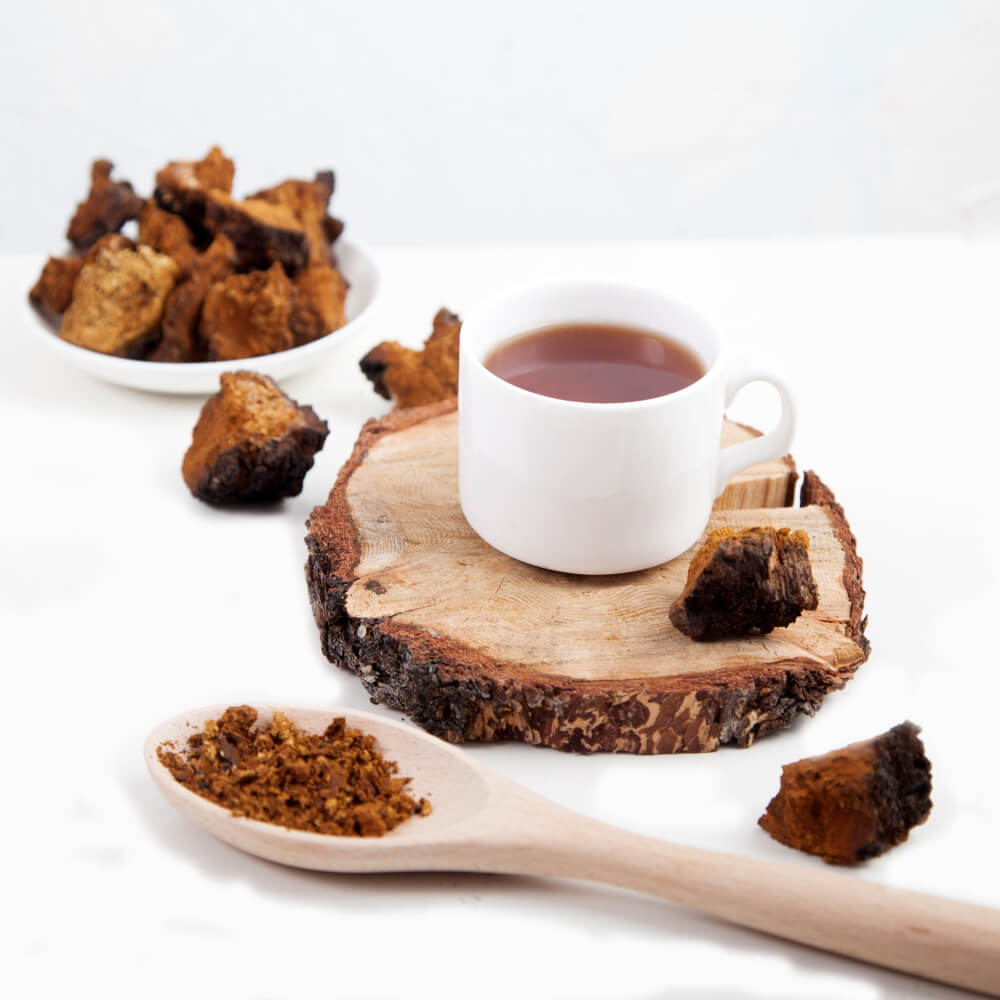In this image, a white mug filled with a brown liquid, presumably tea, sits centrally atop a roughly round, dried wooden tree trunk slice used as a coaster. The trunk piece, about two inches thick, displays rich grain patterns on its surface. Surrounding the mug and coaster, there are multiple brown and black chunks that resemble roasted or dried organic material. To the top left, a small white bowl holds more of these brown chunks. Scattered around are a few additional chunks and some grainy brown material. A wooden spoon, coated with similar brown granules, extends from the bottom right corner, its handle reaching toward the mug. The entire arrangement rests on a clean, white surface, suggesting a minimalistic yet thoughtfully composed setting. The background features a faint glimpse of a light blue or gray wall. The overall color palette includes whites, browns, and blacks, contributing to a natural and serene aesthetic.